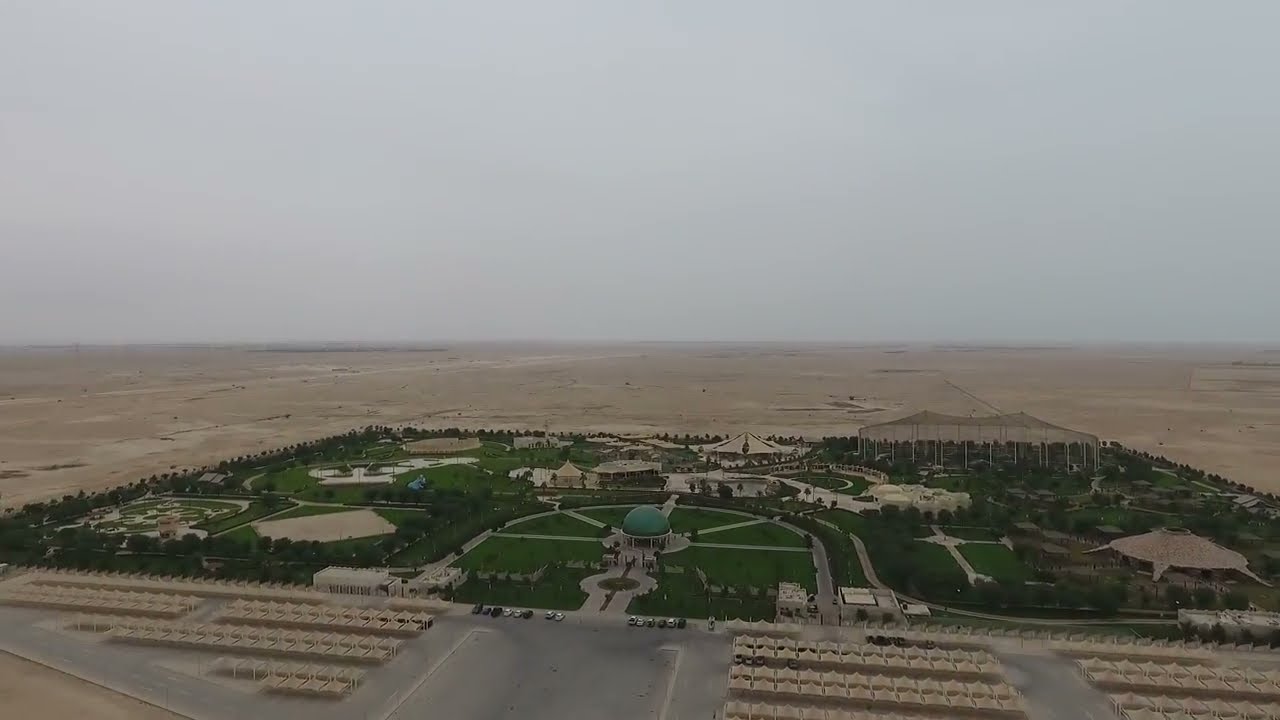This image depicts a detailed, top-down view of a large, rectangular green plot of land that contrasts starkly with the surrounding desert-like, flat, sandy brown soil. The central feature of this area is a lush, green lawn, meticulously maintained, and surrounded by rows of trees along its boundary. Dominating the center is a white building with a blueish-green dome, reminiscent of classic architecture. Leading up to this building is a stone pathway that begins as a rectangle and transitions into a rounded shape closer to the structure. 

Adjacent to this central building, multiple smaller structures are scattered, resembling the size of storage units or small tents, arranged in neat rows. On the far right, there is a larger building with a white top, and directly in front of the green lawn is a road intersecting with additional concrete plots. The bottom section of the green area hosts another significant building, distinguished by its red wall and blue roof. 

In the foreground, there are cars and other smaller unidentified structures, possibly small buildings or storage units. Paths crisscross the green area, connecting the various buildings and sections. The background fades into an expansive desert, extending the barren landscape except for this meticulously cultivated green plot. Above, the sky is a dull, light gray, suggesting an overcast day or evening.